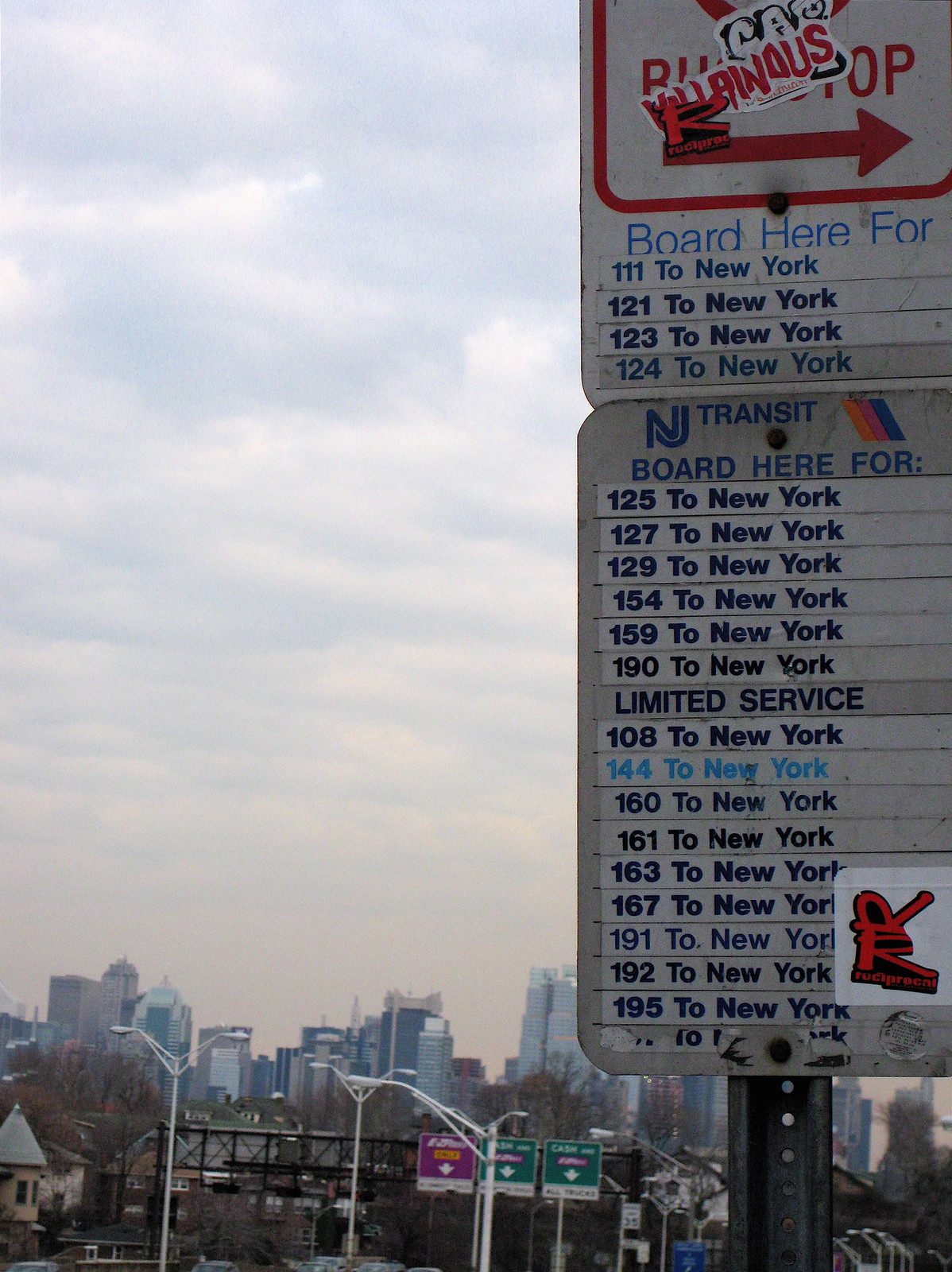The photograph captures a cloudy, overcast day in what seems to be or near New York City. Dominating the background are tall buildings indicating a city skyline. Street lamps are also visible, suggesting that a street runs behind the main subject of the image. In the foreground toward the right, there is a bus stop sign covered with a few stickers. The stickers partially obscure parts of the text, with phrases like "CAP something," "Killinius" in red, and two stylized R's. 

The bus stop sign itself is segmented into three parts. The first section reads "Board Here 4" followed by bus numbers: 111, 121, 123, and 124, all heading to New York. The second section says "NJ Transit Board Here 4" with bus numbers 125, 127, 129, 154, and 159 to New York. The final section, labeled "Limited Service," lists more bus numbers also traveling to New York: 108, 144 (in a lighter blue than the others), 160, 161, 163, 167, 191, 192, and 195. The scene is set against a very cloudy and hazy sky, giving the impression of a gloomy day.